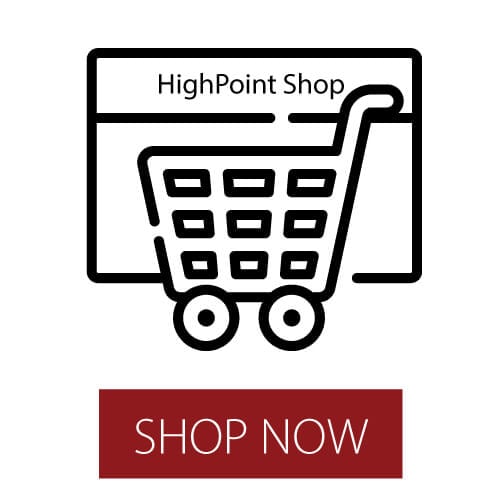This digital image features a simplistic, black-and-white diagram of a shopping cart, prominently displayed with two visible wheels, a handle on the right side, and a basket marked by six square openings, typical of a supermarket cart. Above the cart, the phrase "High Point Shop" is written within a rectangular outline, providing the name of the potential store. Below the cart, a bold red button, with the words "SHOP NOW" inscribed in capital letters in white, beckons viewers to take action. The entire image is set against a stark white background, emphasizing its clean, minimalistic design.